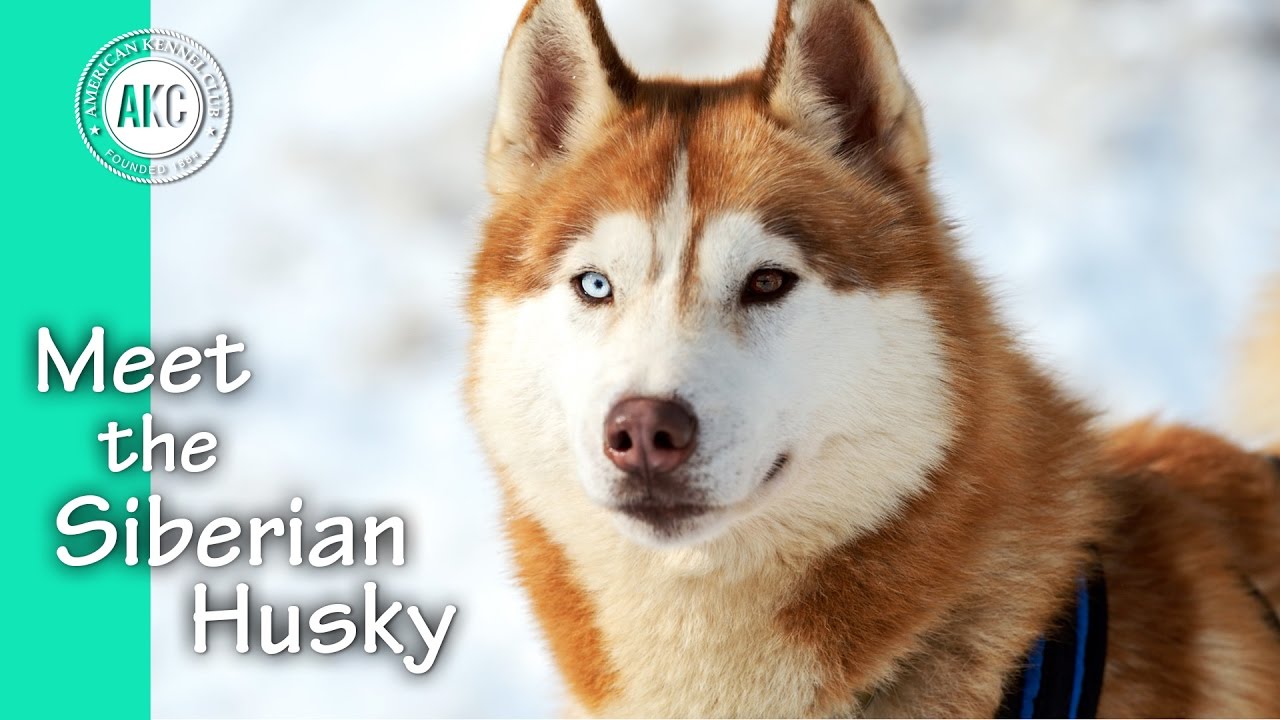The image showcases a striking Siberian Husky facing directly towards the camera, its expressive face fully visible. The dog's eyes illustrate a captivating feature with heterochromia; the left eye exhibits a vibrant turquoise blue while the right eye is a rich dark brown. The husky's fur is predominantly white with a framing of russet-hued fur around the edges of its face, stretching towards its back. The nose is a dark mocha color, giving contrast to its otherwise lighter hues. Adorned with a black and blue-striped leash, the husky's neck and a portion of its shoulder are visible, but its legs are not in the frame.

To the left of the husky, a caption reads "Meet the Siberian Husky," and at the top left corner, the AKC (American Kennel Club) logo is placed, indicating the establishment year, albeit somewhat unclear in two of the descriptions. The background resembles a snowy white landscape, enhancing the pristine and vibrant appearance of the dog. Adjacent to the left edge of the image is a turquoise-green stripe, adding a touch of color to the composition. The setting evokes an outdoor scene, amplifying the natural beauty of this magnificent husky.